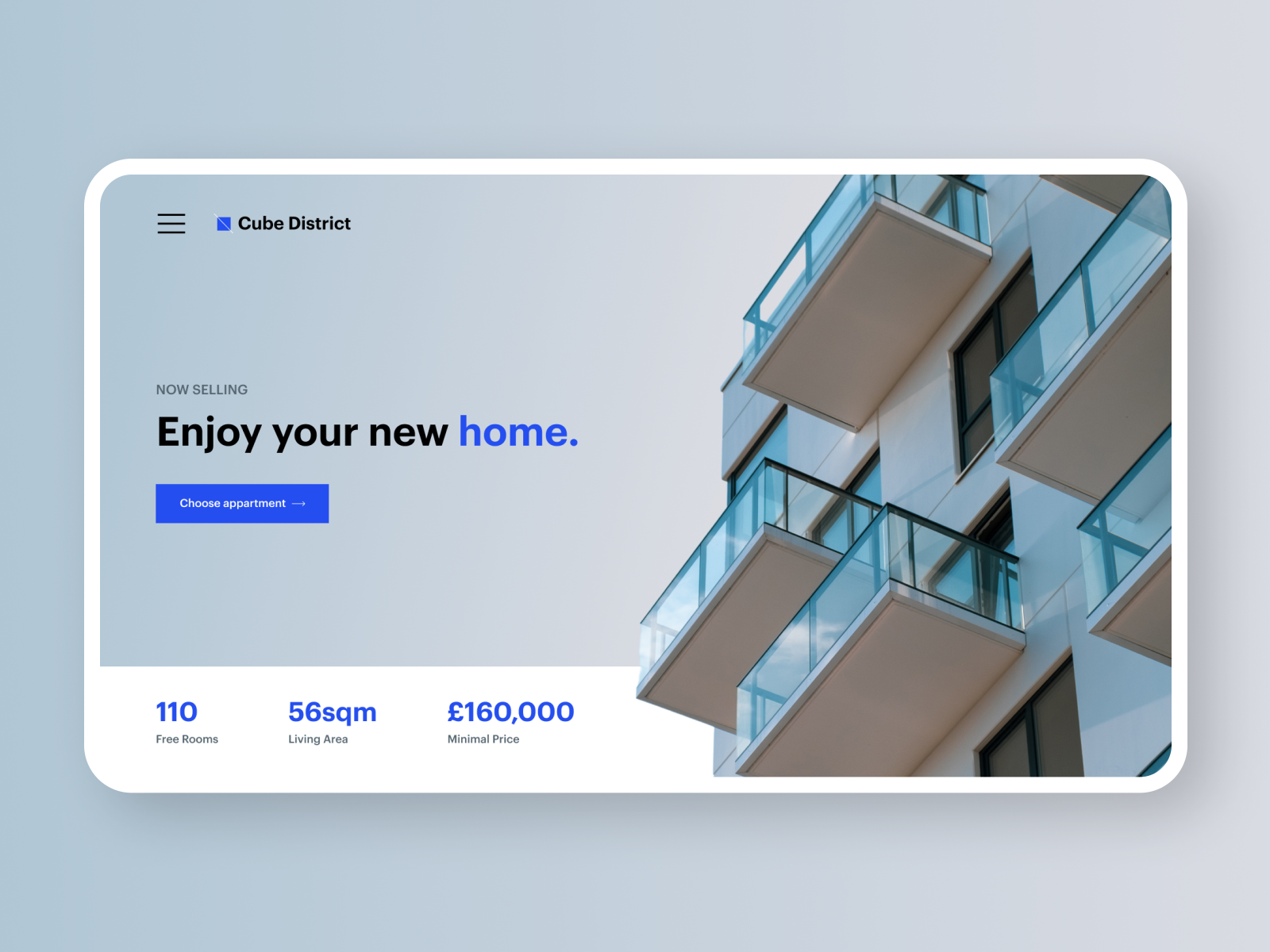This detailed website interface mock-up showcases a real estate project named Cube District. The design emphasizes a clean, modern aesthetic with a primary focus on promoting new apartments for sale. Dominating the background is a close-up photograph of a sleek, contemporary apartment building featuring glass balconies.

Key design elements include:
- **Top Left Corner**: The Cube District logo and name are prominently displayed.
- **Navigation Menu**: Directly below the logo is an icon represented by horizontal lines, indicating a collapsible navigation menu.
- **Main Headline**: Centrally positioned, the headline reads "Enjoy your new home," with the word "home" highlighted in blue for emphasis.
- **Call to Action**: Situated below the headline is a button labeled "Choose Apartment," inviting users to view available options.
- **Bottom Left Corner**: Informational text indicates the number of available units ("110 free rooms"), the living area size ("56 square miles living area"), and the starting price ("£160,000 minimum price").

The overall design employs a minimalist approach, using a white and blue color scheme to exude professionalism and appeal. While visually cohesive and elegant, this design strategy is common in modern web interfaces.